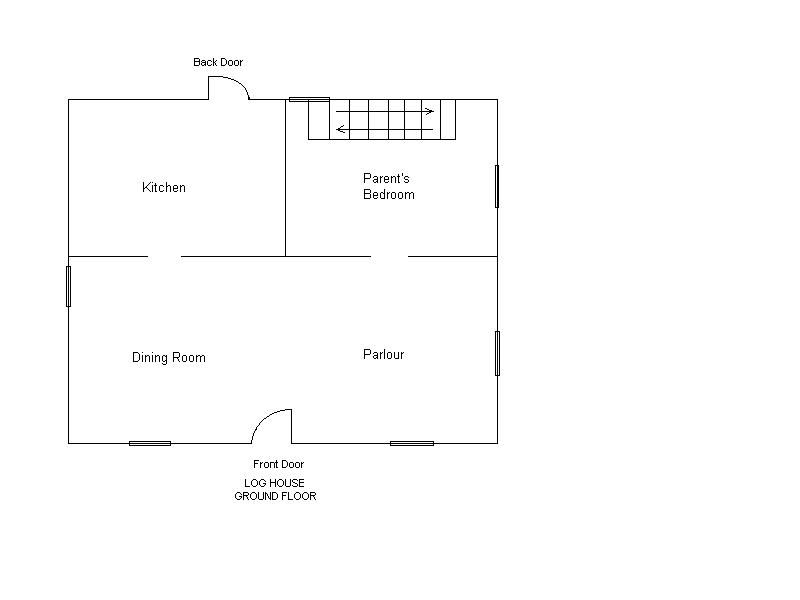Blueprint of the Ground Floor of a Log House:

This blueprint depicts the ground floor layout of a log house, characterized by a simple and clean design. The image shows the front door located at the very bottom, leading into a spacious, open-plan area that combines the dining room on the left and the parlour on the right, without any dividing walls. 

In the top left corner, accessible through the dining room, is the kitchen equipped with a back door that leads outside. The kitchen appears to be windowless.

On the opposite side, through the parlour in the bottom right, is the parents' bedroom, occupying the top right segment of the layout. This room features a single window on the side of the house. 

Additionally, a staircase is situated along the back wall, providing access to other floors. The ground floor boasts two windows at the front, one in the dining room and another in the parlour, along with an additional side window in the parlour.

The plan does not provide measurements, leaving the dimensions of the house unspecified. Overall, the blueprint illustrates a balanced mix of communal and private spaces, emphasizing an open concept for the front portion of the house.